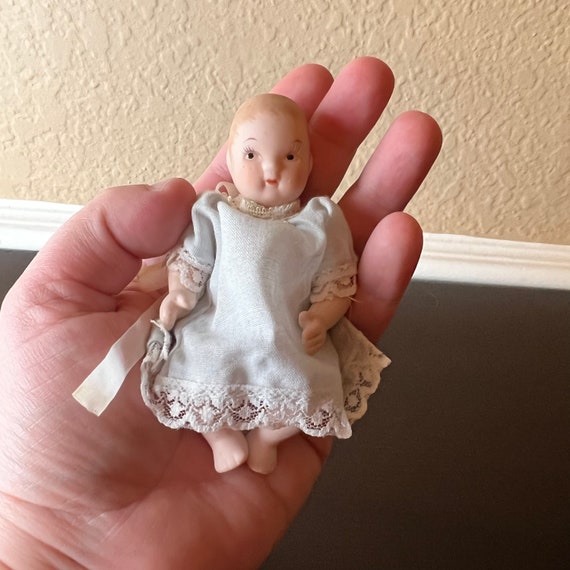This full-color, square photograph captures a left hand, palm up, holding a small baby doll. The scene appears to be taken indoors, likely in someone's home, using natural light. The doll, resembling a baby, wears a white gown that covers it from neck to toe, with visible arms and feet protruding from the gown. The doll's features include blonde hair and a small mouth.

The background features distinct elements: the lower half is a dark, possibly black wall, transitioning above a white crown molding to a textured beige upper wall. This textured wall, which visually dominates the upper third of the image, would feel rough to touch. The hand holding the doll appears pudgy, suggesting it might belong to a child, adding a tender and intimate perspective to the photograph.